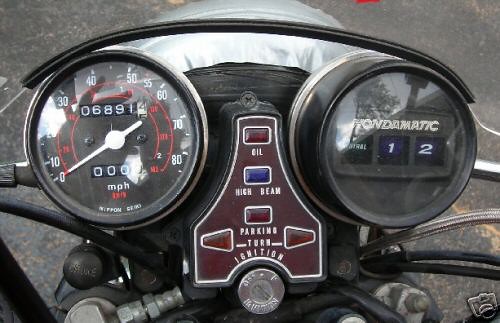The image showcases the dashboard of a motorcycle, captured from a straight-on perspective. Prominently featured are two round gauges: a speedometer and another gauge that measures a different parameter. The odometer on the speedometer displays a mileage of 6,891. The backgrounds of these gauges are black, with white numbers for easy readability.

The speedometer includes a striking red half-moon shape, which immediately draws the eye to the speed readings. Through the tangle of wires connecting the motorcycle's components, the road ahead is faintly visible.

Additional indicators on the dashboard include an oil gauge, a high beam indicator, parking turn signal indicators, and the ignition switch where the key is inserted. There are silver connections attached to these wires, adding to the intricate details of the dashboard's layout. In the background, part of the motorcycle's metallic frame is visible, hinting at either a fender or another component. The image gives a detailed and comprehensive view of the motorcycle's instrument panel and surrounding elements.